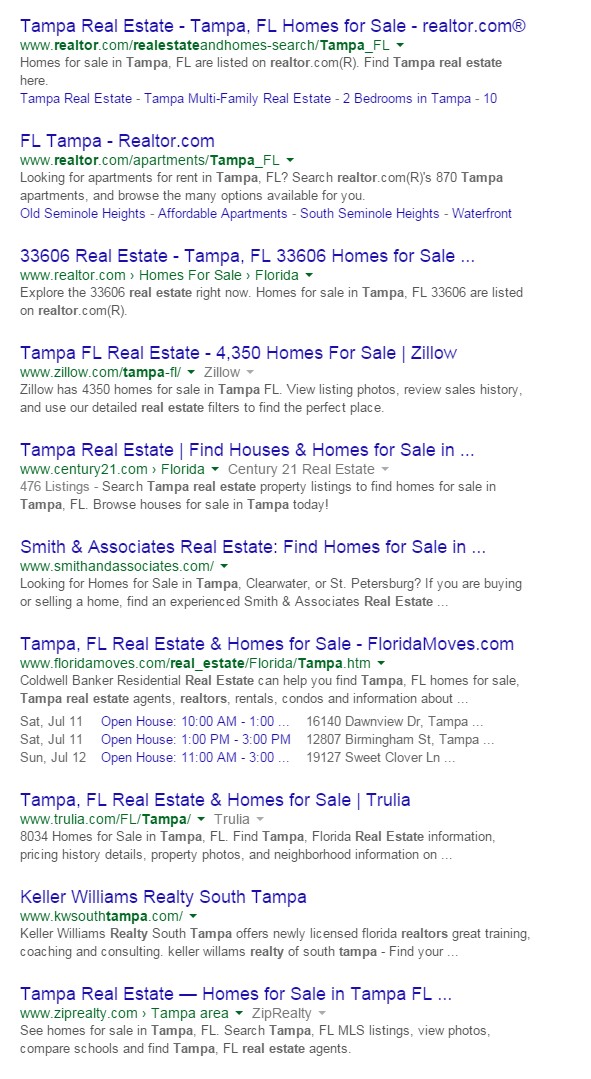The image showcases a screenshot of Google search results for real estate in Tampa, Florida. The image is notably taller than it is wide, with no discernible background aside from the light emanating from the computer screen, which illuminates the search results clearly. Though "Google" is not explicitly mentioned, the layout is unmistakably that of Google search results.

The screenshot reveals a list of ten search listings. The search results are organized in the typical Google format, where the title of each listing appears in blue, the website URL is displayed in green, and the brief description beneath the title is in black text. Additional links within the descriptions, also in blue, provide more navigation options.

The top listing is for "Tampa Real Estate" with a URL from realtor.com that reads: "www.realtor.com/realestateandhomesearch-Tampa_FL." The following listings include "FLTampaRealtor.com" and "33606 Real Estate, Tampa, Florida," among others.

From the content of the search results, it is evident that the user is searching for real estate agents or listings in Tampa, Florida. Recognizable names like Trulia, Keller Williams, Century 21, and Zillow appear among the results, suggesting that the search was intended to find a reliable realtor or real estate listings.

The dimensions and layout of the image imply it was likely taken from a computer screen rather than a mobile device, helping to provide a comprehensive view of the entire search result page. The user's focus on multiple real estate-related search results indicates a clear intent to find real estate services or homes for sale in the Tampa area.